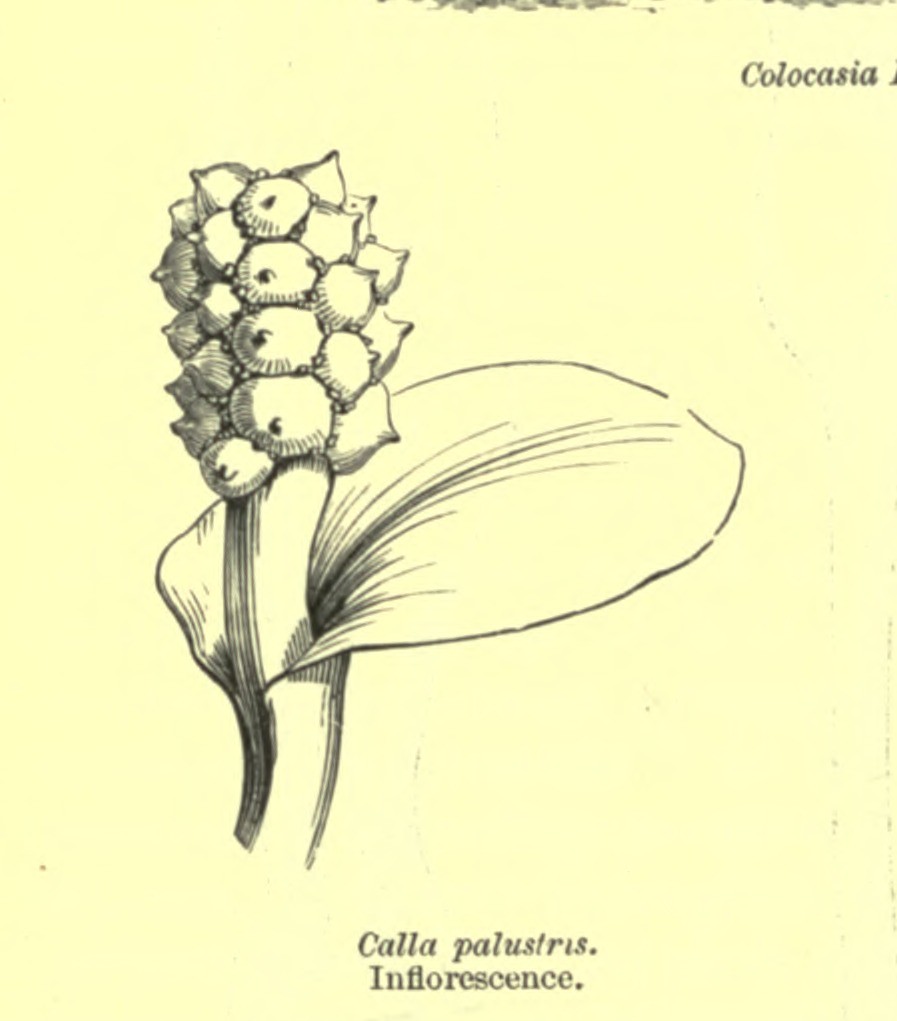This illustration features a detailed black ink line drawing set against a pale peach or beige background, resembling an excerpt from a botanical book or magazine. The central focus is a plant characterized by a single broad, oval-shaped leaf and a thick, prominent stem. Along this stem, clusters of circular, pointed structures, resembling small onion-shaped pods or teats, are arranged vertically in rows of four or five, hinting they might be seeds or immature flowers. Below the illustration, the italicized Latin name "Cala palustris" appears, followed by "inflorescence" in regular font. In the upper right corner, a partially cut-off italicized text reads "Colocasia," surrounded by sketch marks that add an artistic, hand-drawn feel to the image.